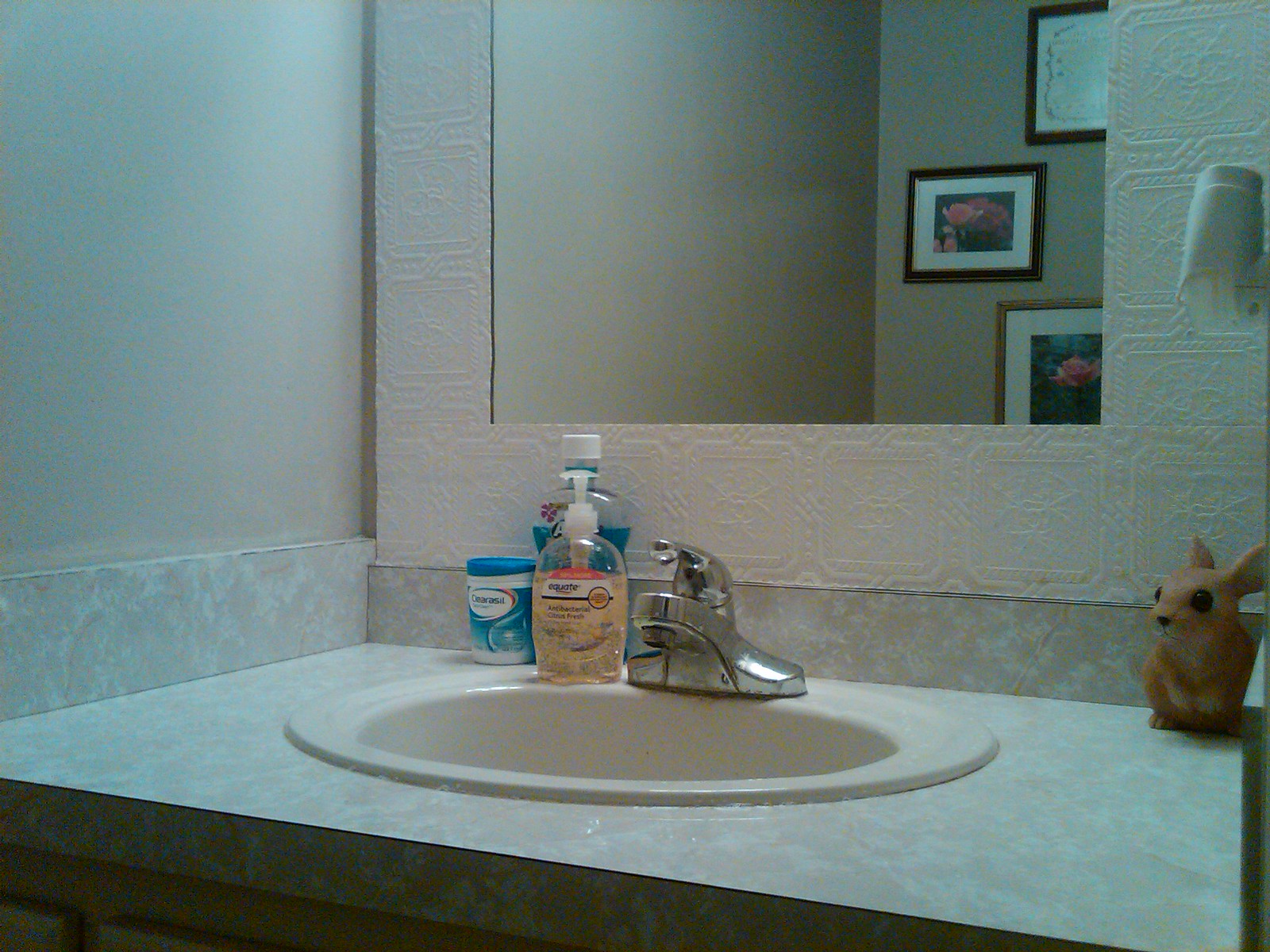This photograph, slightly wider than it is tall, captures a detailed view of a bathroom. The composition is angled as if the camera is positioned slightly to the right, giving a diagonal perspective towards the left. At the focal point is an oval-shaped sink with a nickel-colored faucet, positioned just below the center and slightly to the left. Embedded in the wall above the sink is a mirror reflecting part of the bathroom's interior.

To the right of the sink, against the wall, stands a small sculpture of a bunny rabbit, serving as a charming decorative piece. The sink area is neatly organized with three dispensers: one labeled 'Equate' which appears to be hand soap, another labeled 'Clearasil', and a third dispenser, filled a little more than three-quarters with blue liquid, likely mouthwash, identifiable by the partially visible letter 'A' on the container.

In the reflection within the mirror, three pictures are visible on the opposite wall: the bottom two displaying floral images, while the subject of the top one remains unclear. The entire image possesses a slight bluish tint, suggesting an undersaturation with hues subtly shifted towards blue. Additionally, visible above the bunny sculpture on the right side, there appears to be either a sconce or an air freshener plugged in, contributing to the overall ambiance of the bathroom.